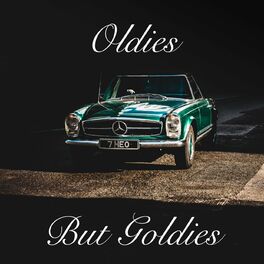The image is a small, dark, square photograph featuring an older model green or turquoise Mercedes-Benz. The majority of the background is black, with the car illuminated slightly in the center. The Mercedes is positioned facing the viewer, displaying a silver front grille, round headlights, and a European-style black rectangle license plate with a silver frame, bearing the number 7HE0. The vehicle, possibly a coupe or convertible, features silver accents down the sides, including door handles and rims to match the black tires. There is a radio antenna on the passenger side front. The car is set against what appears to be a tile or roadway, with a brown hue to the ground. Above the car, the black background features the words "Oldies" in white cursive script, and below, in an identical script, it says "but Goldies," highlighting the timeless appeal of the classic vehicle. Light is shining on the car from the right, emphasizing it against the dark surroundings.